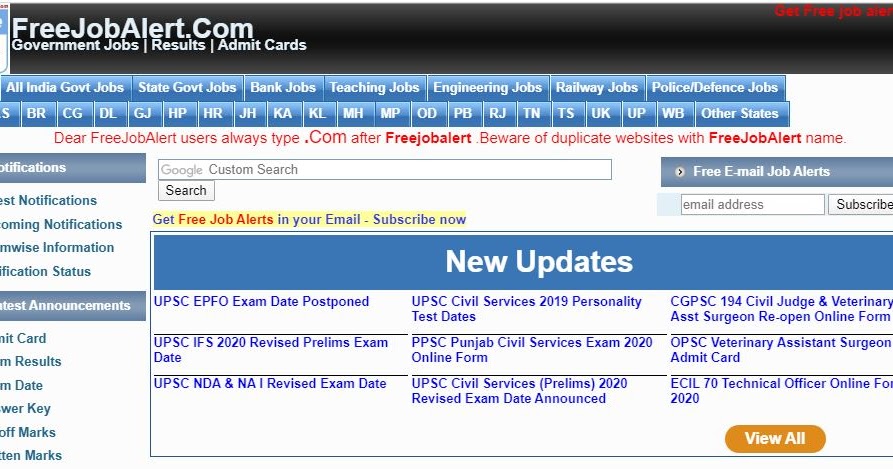Screenshot of the FreeJobAlert.com website, showcasing a cluttered and poorly designed user interface. The site’s name is prominently displayed with the letters "F," "J," "A," and "C" capitalized, and the tagline "Government Jobs, Results, and Admin Cards" just below. A navigation bar follows, featuring various job categories such as All India Government Jobs, State Government Jobs, Bank Jobs, Teaching Jobs, Engineering Jobs, Rail Jobs, and Police and Defense Jobs. Beneath the menu, a list of states abbreviated with letters like B, R, C, G, D, L, and more spans across the screen. A bold red warning advises users to type ".com" after FreeJobAlert and cautions against duplicate websites.

A Google Custom Search field is located below the warning. On the left side of the screen, partially obscured menu options suggest additional functionality, including an alert subscription feature where users can enter their email addresses for updates. The main content area displays various updates, such as UPSC EPFO exam date postponements and UPSC Civil Services 2019 personality test dates, organized in nine detailed entries. Notably, PPSC Punjab Civil Services exam 2020 online form is highlighted. To the right, a conspicuous brownish mustard-colored button labeled "View All" invites further exploration. The site appears to cater specifically to users in India.